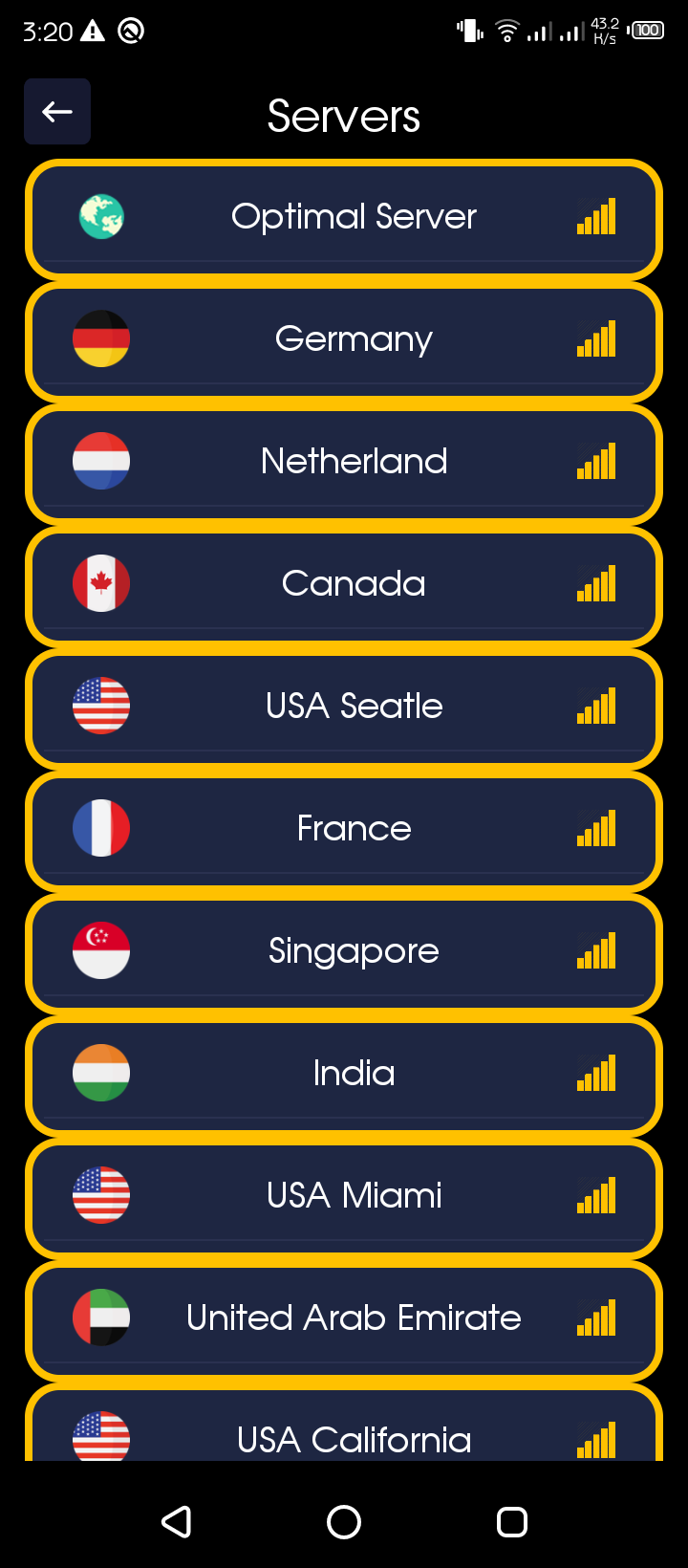A highly detailed photo captured from a cell phone screen shows a server selection page. The background is predominantly black, with the top section featuring a navy-colored bar framed by yellow rectangles. At the very top, the time reads 3:20, and various icons are displayed, including Wi-Fi signal strength, cellular bars, and a reading of "43.2 H/S". The battery icon shows 100%, indicating a full charge.

Below this top bar, the page is titled "Servers" with a left-pointing arrow. As you scroll down, there is an image of a globe labeled "Optimal Server" followed by several yellow bar graphs arranged vertically, with each bar fully filled.

Moving further down the page, the first section displays the flag of Germany in black, red, and yellow. Next is the Netherlands with a flag of red, white, and blue. Following are Canada's flag with its distinct red maple leaf center, the US flag indicating Seattle, France's tricolor flag, Singapore, India's tricolor flag with the Ashoka Chakra, another US flag this time for Miami, the flag of the United Arab Emirates, and lastly, a US flag for California.